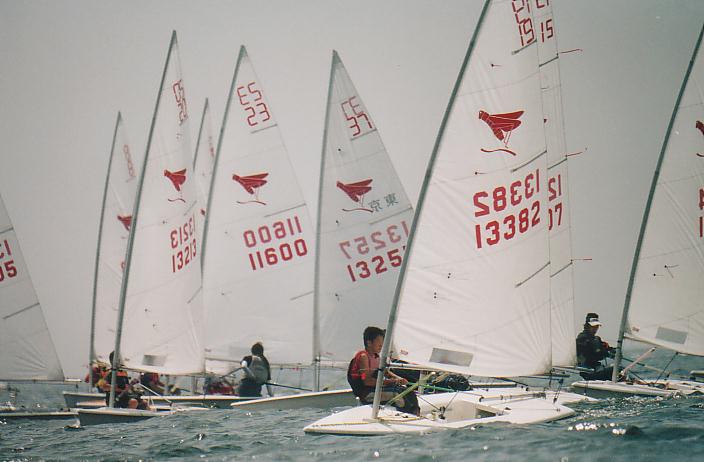The image depicts a serene scene on the ocean, featuring roughly ten small sailboats with white sails, each adorned with distinctive red numbers for identification. Each sail is marked with a red kite-like symbol or possibly a grasshopper, suggesting a common affiliation, likely indicating a sail school or a team. The water beneath them is clear and blue, and various figures can be seen manning the boats, mostly young individuals who might be participating in a water sports competition or a sailing activity holiday. Among the sailors, a mix of youthful participants and possibly an instructor are visible. The sails are tall and predominantly white, embellished with red writing and numbers, while beneath the main symbol, there's a blank white space. The overall atmosphere suggests an organized, competitive, or training event set against the backdrop of calm waters.